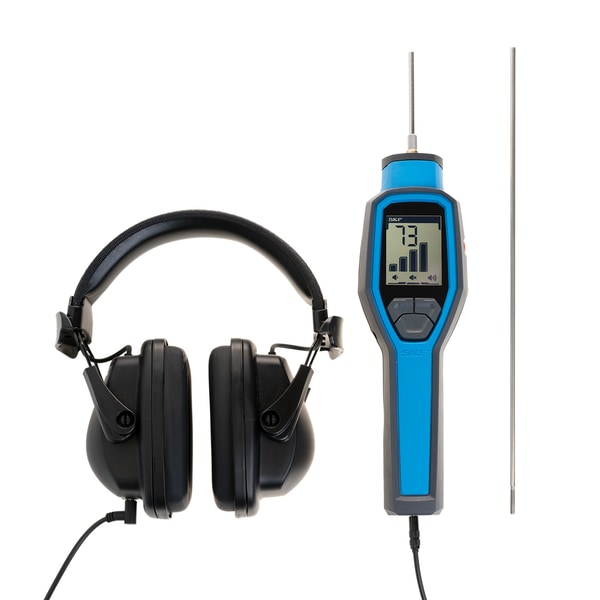The image displays a product layout against a white background, suitable for an e-commerce platform like Amazon or Walmart. On the left side of the image, there is a set of black wired headphones. These headphones feature large, rubberized foam ear supports and a cushioned head strap for comfort. Metal straps connect the ear cups, which also have a jack on the bottom left side. Adjacent to the headphones is a blue measuring device with a gray shell. This device has an electronic screen displaying the number 73 and includes a four-bar chart indicator. It is equipped with three grey buttons on the front and has a wired connection that appears to lead to a metallic stick-like tool positioned on the far right of the image. The detailed layout and distinct features of both items suggest they are part of a professional audio or measurement set.